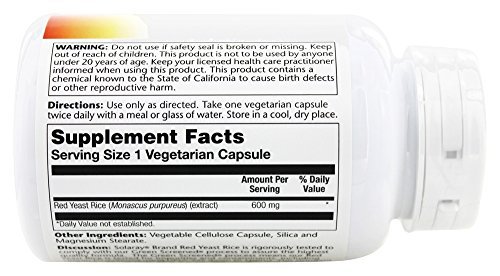This image is a close-up of a white plastic supplement bottle with a matching white cap, positioned on its side. The primary focus is on the back label of the bottle, which details various important information. The visible sections of the label include usage directions, warnings, and supplement facts. The bottle's front label is partially visible, showcasing a design that transitions from orange to yellow and finally to white.

The warnings on the label specifically caution against using the product if the safety seal is broken or missing. It also advises keeping the bottle out of reach of children. A notable warning states that the product contains a chemical known to the state of California to cause birth defects or other reproductive harm.

Usage directions are clearly outlined, instructing users to take one capsule twice a day, ideally with a meal or a glass of water. The supplement facts reveal that the primary ingredient in the product is Red Yeast Rice, with a dosage of 600 milligrams per capsule.